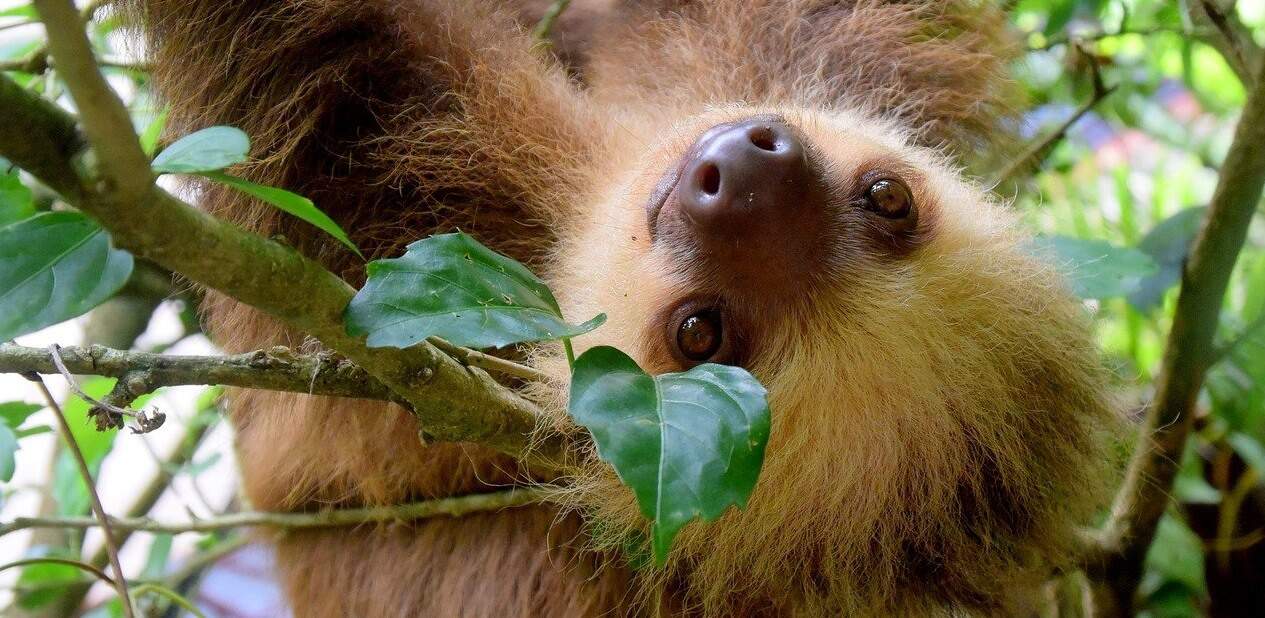The photograph captures an extremely close-up view of a sloth, hanging upside down in a tree. The sloth's furry face, featuring a mix of light golden, dark brown, and lighter white-yellow fur, takes up about 80% of the frame. Its wide, brown eyes and dark brown nose, which some describe as having a dark purple hue, are prominently visible, giving the sloth almost a smiling expression. The sloth appears to be young and very fluffy. Surrounding the sloth is a setting of foliage and various tree branches. A large stick extends from the top left to the center of the image, with five green leaves attached. Additional deep green leaves, along with greenish brown branches, are visible in the background. There's also a noticeable light source coming from the bottom left and top right corners of the image, suggesting it was taken during the daytime, with some parts of the background appearing blurry, enhancing the focus on the sloth.